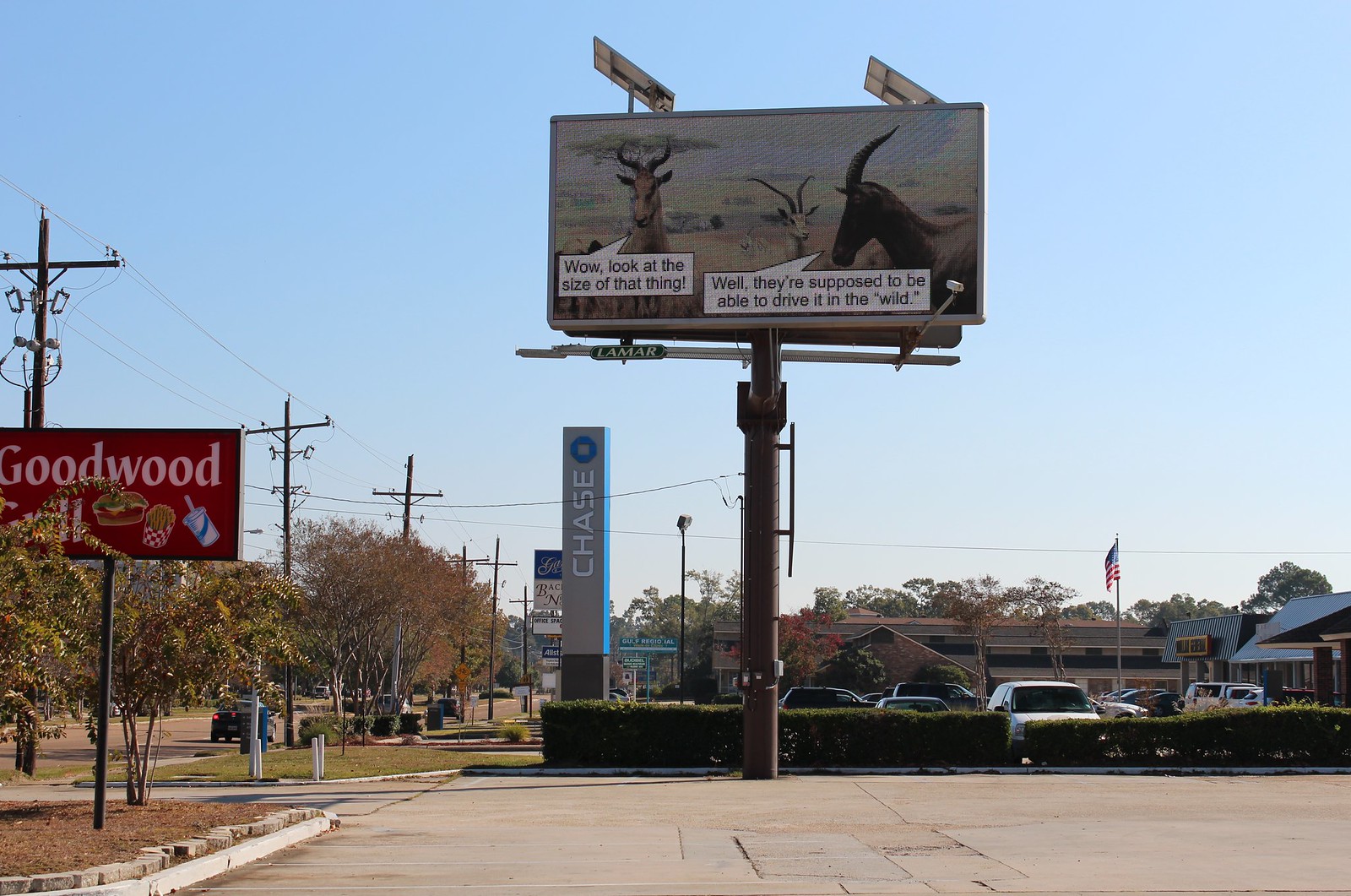The photograph captures an outdoor billboard set against a clear, blue sky. The billboard is prominently positioned in the center, supported by a sturdy metal pole. The billboard itself is rectangular and features what appears to be a painted image of an African landscape, complete with a blue sky and three animals that resemble antelopes or caribou. These animals are brown and white with indistinct antlers. Beneath two of the animals are white text boxes with unreadable black lettering, appearing as if the animals are saying something.

Flanking the main billboard are two smaller signs. On the right, there's a vertical sign for Chase Bank, featuring a blue and white design with the bank's logo and lettering arranged counterclockwise. On the left, there's a 'Goodwood' sign set against a red background decorated with icons of food items like drinks and pizza. This smaller sign is attached to a black pole.

Below these billboards lies a parking lot, partially obscured by cement surfaces and shrubbery. Some cars are visible on the right side of the image, though they are mostly hidden behind the greenery. The overall scene merges urban elements with a touch of natural beauty, providing a vibrant snapshot of the area.